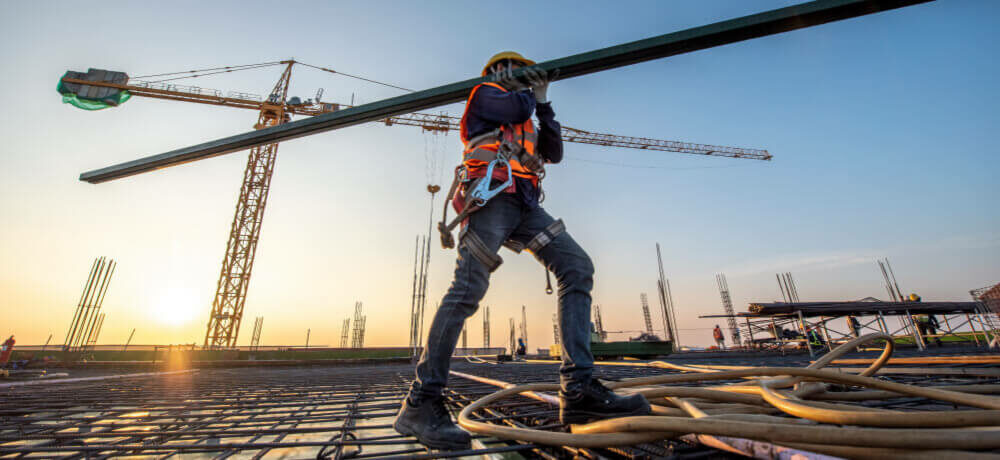In this nearly panoramic image taken in the morning, a construction worker, identifiable by his orange safety vest, blue jeans, black boots, and yellow hard hat, is captured mid-stride as he carefully navigates across a network of rebar. He is carrying a long, steel bar on his right shoulder and is beginning to step over a thick, beige hose situated in the bottom right corner of the frame. The camera angle from below accentuates the worker's focus and the intricate web of rebar beneath him. The morning sun casts an orange glow on the left side of the sky, gradually blending into shades of blue towards the top and right. In the background, a towering crane looms, hinting at the future construction of what will likely be a high-rise building. Additional workers can be seen in the distance amidst various metal scaffolding and protruding rebar, all set against a broad expanse of sky.